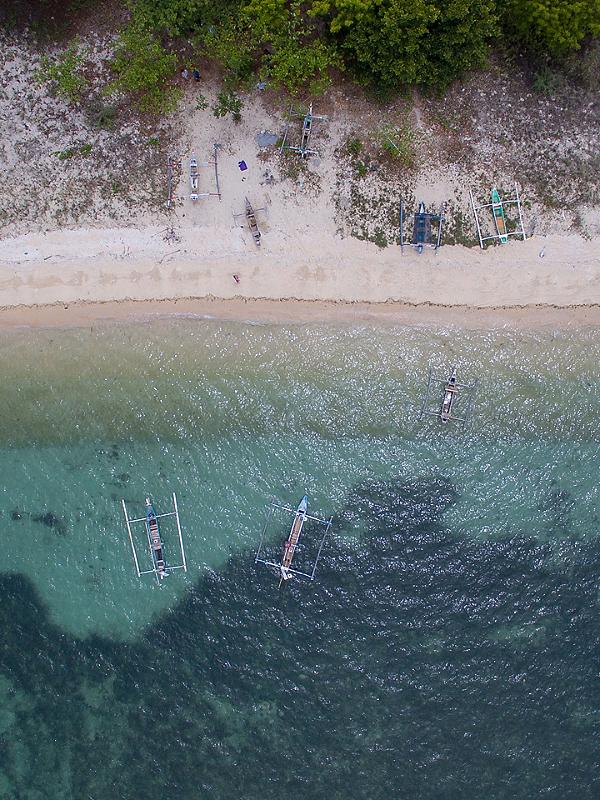This is an aerial view of a tranquil ocean area with a sandy beach. The bottom half of the image showcases the crystal-clear water shifting in color from dark blue to light blue as it approaches the shore. The water is calm and glistens with sunlight, revealing a greenish hue in the shallows where the sand is visible underneath. In the water, there are three unique vessels; they appear to be catamarans or similar, each with distinctive rectangular structures on their sides. These vessels, anchored and empty, mirror five more identical ones lined up on the light-colored sandy shore. The beach itself transitions from sand to areas with small patches of foliage, leading up to a dense row of green trees at the top of the image. In this serene scene, only three people are visible near the line of trees, adding a subtle touch of human presence to the otherwise peaceful coastal landscape.